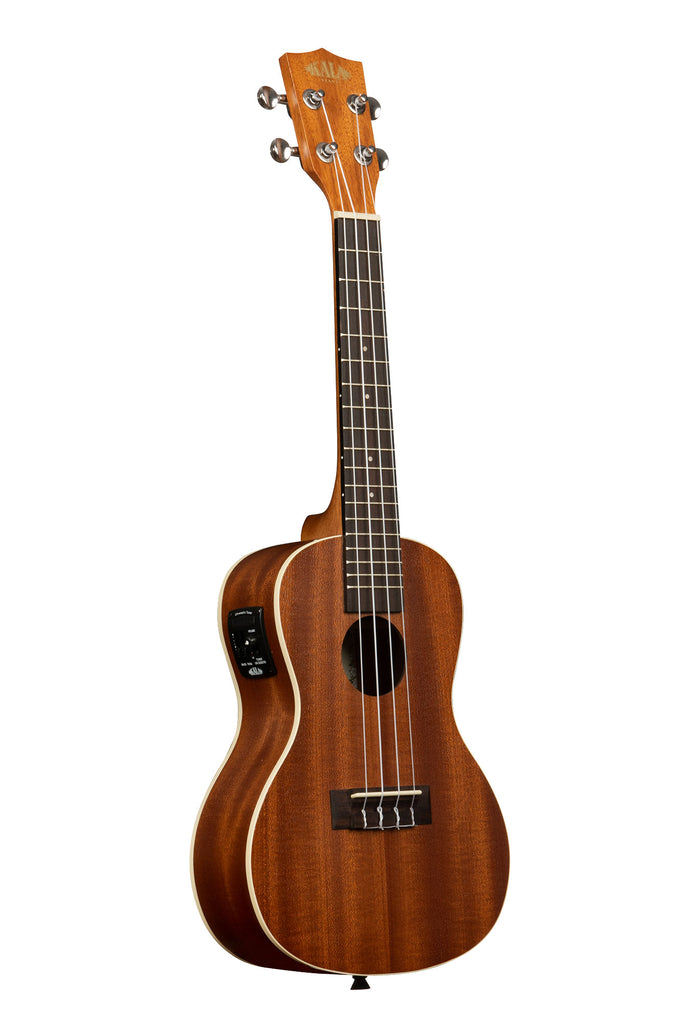This image depicts a small, possibly ukulele-like, string instrument against a white background, reminiscent of a product photo. The instrument, identified as a Kala ukulele, features the brand name "Kala" in gold lettering atop its light brown headstock. The tuning pegs, four in total, are silver and positioned at the headstock to adjust the tension of the white strings that extend down a black fretboard adorned with white stripes. The body of the ukulele is dark brown with a fine wood grain, accented by a slim off-white binding that runs around its edges. In the upper middle of the body is a central sound hole, characteristic of acoustic instruments. Below the sound hole sits a black bridge with a white saddle, where the strings are anchored. There is a small knob at the bottom of the body for attaching a shoulder strap. The right side of the instrument features a black panel, suggestive of an electric component, which hints at the possibility of this ukulele being an electro-acoustic model. The overall design is traditional, with a narrower top curving into a wider lower section, generating a classic, yet refined appearance.